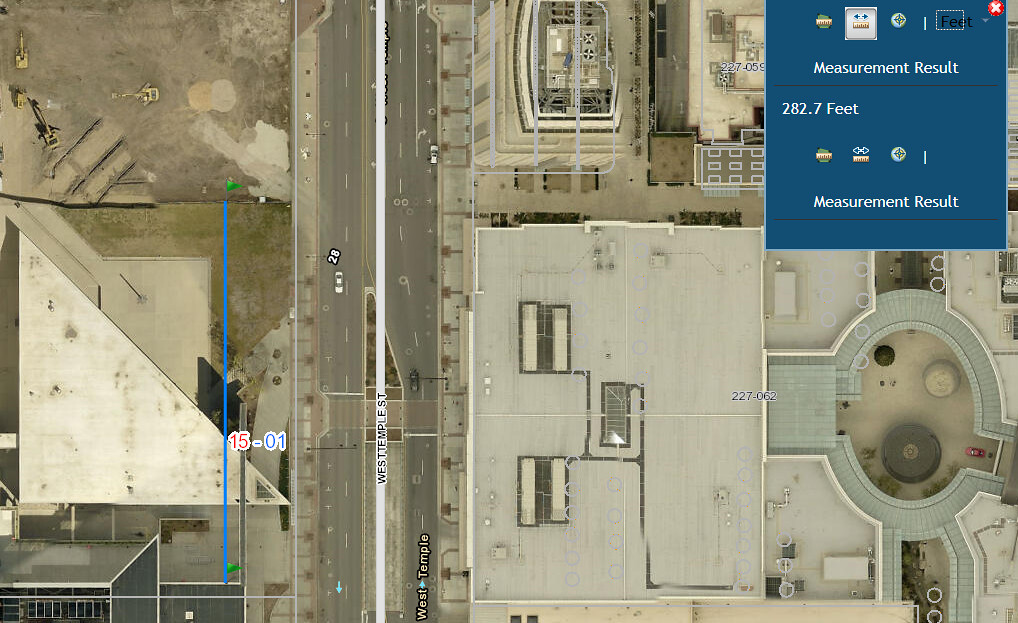This satellite image provides an aerial view of an urban area, showcasing various landmarks and measurement results. 

At the top right of the image, there is a prominent blue square labeled "Measurement Result." Inside this blue square, different measurement tools are illustrated. The first tool is represented as a small green circle with a ruler inside. The second tool is a large white square with a ruler and two plus signs above it. The third tool is depicted as a tiny dot with a target symbol. To the right of these tools, the text "Feet" is written in black, with "282.7 feet" displayed in white text within the blue square.

On the bottom left of the image, a vertical blue line marked "15-01" extends slightly to the right and goes upward, dividing a plot of land. This area includes a triangular building with a visible rooftop. The top left corner of the image features a large dirt field, while the central part is intersected by a two-lane road running north and south, labeled "West Temple Street."

At the top right, there is a tall building with its rooftop and air units visible, primarily in shades of gray. The building's rooftop is also marked with some text, "227.062," in black. Another significant structure is observed at the bottom right; it is a large building composed of four distinct squares.

Additionally, there is a plaza located at the very right of the image, which appears to be made of dirt, stone, or concrete. A red car is parked within this plaza. The plaza also has decorative elements, with half-circles formed from numerous gray rectangles, creating a curved pattern at both the top and bottom of the area.

Overall, the image is characterized by grayscale tones with minimal color variation, providing a detailed yet somewhat monotone overview of the urban landscape.